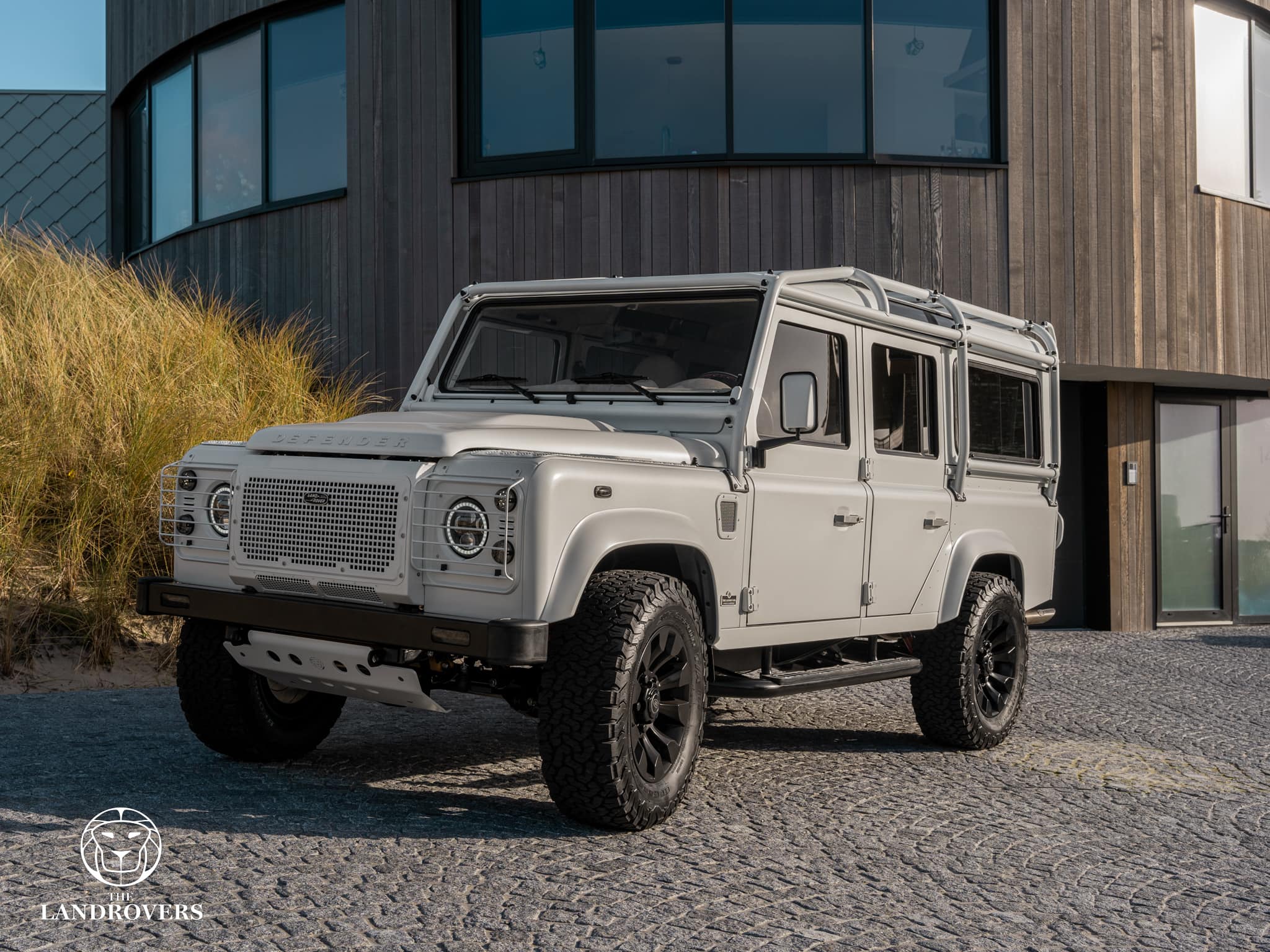This is a detailed photograph of an all-gray Land Rover, distinctly designed for off-road adventures, characterized by its sporty, four-door structure and equipped with black tires. The vehicle, built with light gray steel and featuring a fine mesh grille with chrome horizontal guards across the headlights, stands prominently as the central focus. The two circles in front serve as headlights, and black side steps facilitate easy entry. The Land Rover is parked on a gray cobblestone driveway, oriented diagonally to the left side of the image, which allows a partial view of the front and side windows.

In the background, a modern, two-story, curved wooden building constructed from distressed wooden planks is visible. This building, adorned with a horizontal row of vertical windows trimmed in black on its second floor, adds architectural interest to the scene. In front of the building, on the left side of the image, stands a tall, wispy green bush, nearly the same height as the Land Rover.

The photo was taken during the daytime, with a blue sky noticeable in the upper left-hand corner. At the bottom right of the image, a logo stating "The Land Rovers," accompanied by a circular symbol, can be seen. This detailed setting combines the rugged elegance of the Land Rover with the contemporary design of the wooden building, creating a harmonious yet dynamic composition.